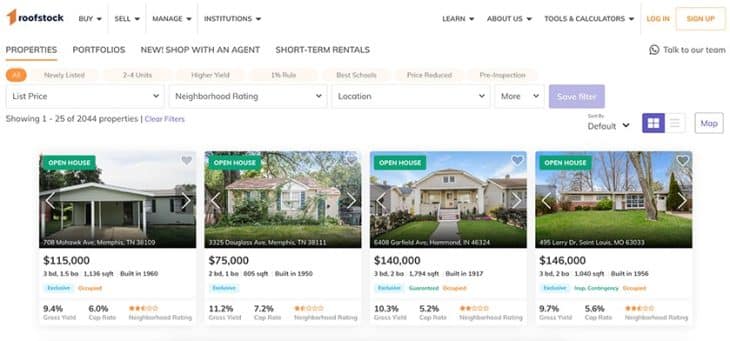The image depicts the homepage of Roofstock.com, a real estate website. In the upper left corner, the logo consists of a red numeral "one" followed by the company name "Roofstock" in black lettering. The top navigation bar features several drop-down menus labeled: "Buy," "Sell," "Manage," and "Institutions." To the right, additional menus such as "Learn," "About Us," and "Tools and Calculators" are available. Further right are links for "Log In" and "Sign Up," beneath which there's a "Talk to Our Team" link for immediate contact.

On the left side of the page, users have access to links for "Properties," "Portfolios," and new offerings like "Shop with an Agent" or "Short-Term Rentals." Scrolling down, detailed links are provided for viewing various property categories such as "All Properties," "Newly Listed," "Two to Four Units," "Higher Yield," "1% Rule," "Best Schools," "Price Reduced," and "Pre-Inspection Homes." In the current view, the "All Properties" filter is applied.

The page includes drop-down filters for refining searches by "List Price," "Neighborhood Rating," "Location," and additional criteria categorized under "More." Users can save their filters and currently, it shows 1 to 25 of 2,044 properties. There's a prominent "Clear Filters" option, and sorting functionalities are provided to organize properties. A map view is also available for geographical search. At the bottom, the page displays images of various properties along with key details such as price, number of bedrooms, and other relevant information.